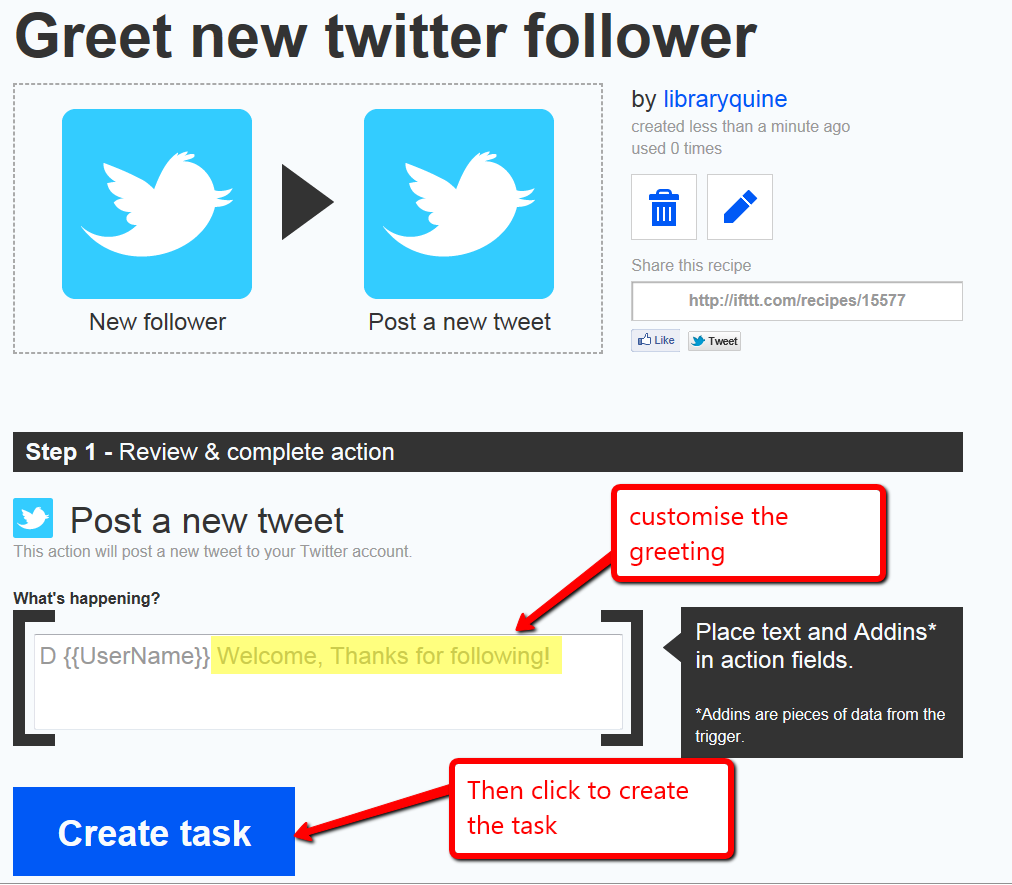The image is divided into two main sections on a white background. At the top, in black text, it reads "Greet new Twitter follower." Below, there is a rectangular box featuring the Twitter logo – a square with a blue background and a white bird. To the right of this square is the text "new follower." A black, right-pointing triangle follows, indicating the progression to the next step: "post a tweet," with the Twitter logo displayed again below this phrase.

Further to the right, the text "by Library Quinn" appears, noting that the task was "created less than a minute ago" and "used zero times." Nearby, icons of a trash can and a pencil offer options to delete or edit the task, respectively. Below, a prompt encourages users to "share this recipe with a website posted."

A black banner underneath this section announces "Step One: Review and complete action." Below this banner, instructions for "Post a new tweet" are illustrated with graphics, guiding users on how to compose a tweet. A text field labeled "what's happening" is surrounded by black brackets, exemplifying an input area where a username and a welcoming message, "Welcome, thanks for following," can be inserted. 

Additionally, a red square highlights the customizable greeting option. To the right of this text box, details on placing text and incorporating add-ins are provided; add-ins are described as pieces of data from the tagger. Finally, at the bottom left corner, a blue button labeled "Create Task" is noted, accompanied by a red square and an arrow pointing towards it, indicating users should "then click to create the task."